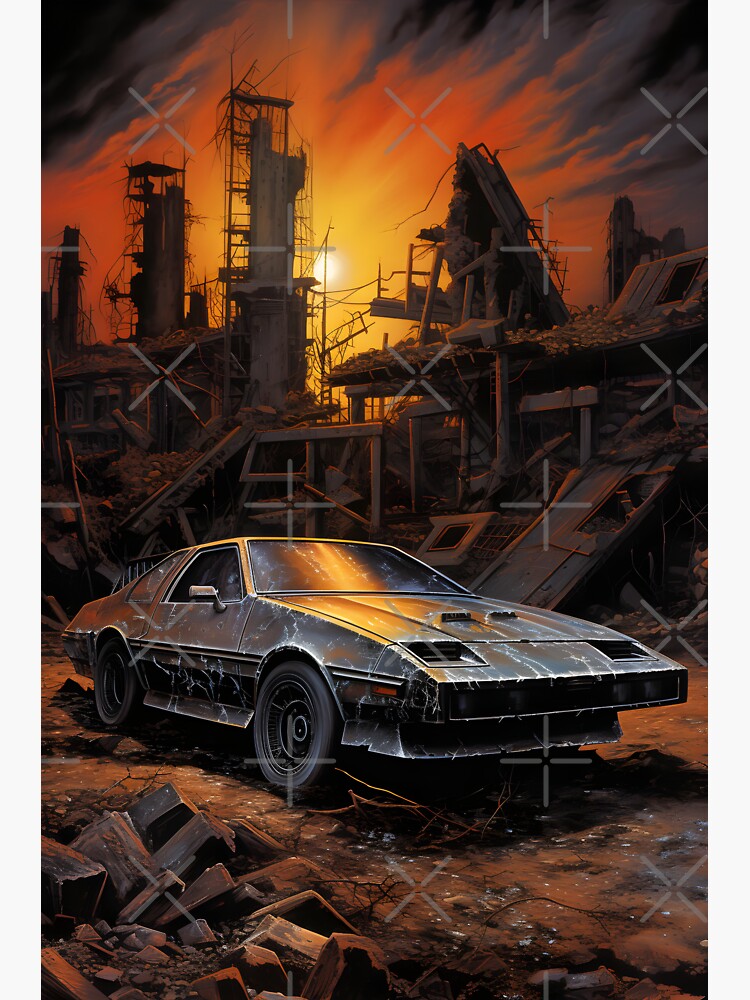The illustration depicts a dystopian, post-apocalyptic scene dominated by the ruins of a factory and a heavily damaged, rusting car that resembles a sports car with squared-off front fenders, possibly reminiscent of a DeLorean, Firebird, or Corvette. The car, though still possessing full tires, is covered in peeling paint and rust, adding to the overall sense of decay. The foreground and the background are strewn with rubble and broken bricks, creating a chaotic environment. The sky, an ominous blend of black, gray, orange, and yellow hues, features a light source that casts an eerie orange fog, suggesting either a perpetual twilight or a world engulfed in flame. The whole scene is veiled with numerous X-shaped watermarks, indicating the image's copyrighted nature, further contributing to its unsettling and desolate ambience.